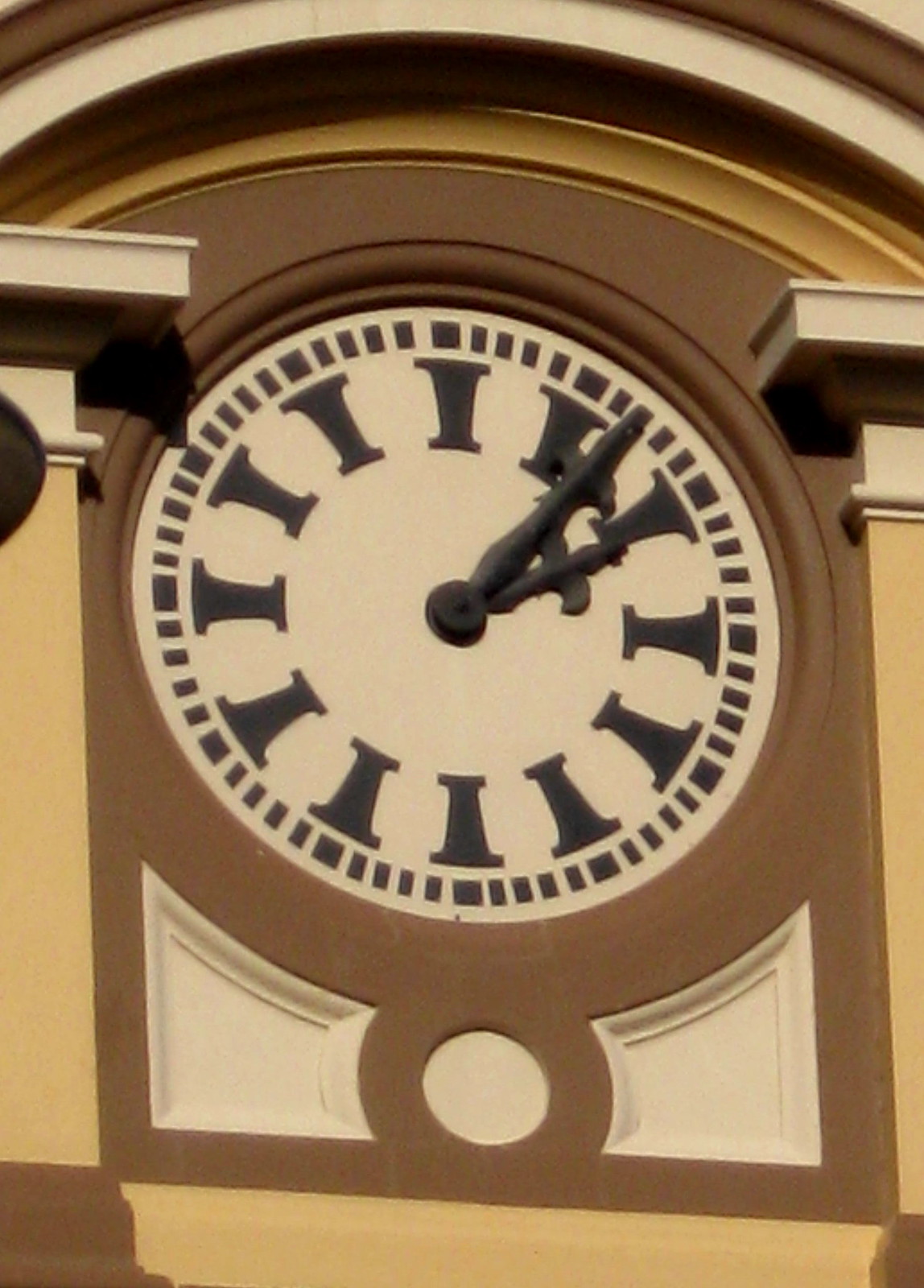The image features a round clock with black hands, displaying a time of approximately 2:06. The clock's face is cream-colored, and instead of numbers, it uses lines to indicate the hours, with smaller lines along the exterior edge. The exterior of the clock is bordered by a brown, stucco-looking material. The clock appears to be mounted on the outside of a tan building. This building features an architectural design with two white-trimmed pillars on either side of the clock and an arch above it. The walls around the clock have a brownish-yellow hue, with white trim accentuating the upper part of the structure. Overall, the scene evokes the facade of a building, possibly resembling a church.